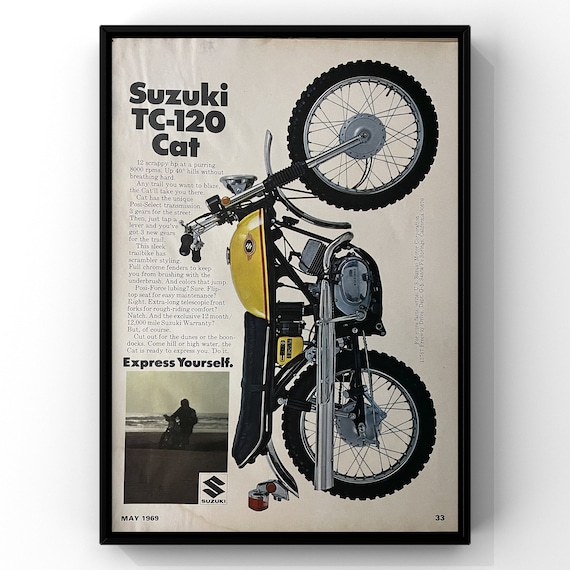The framed image is an advertisement for the Suzuki TC-120 Cat motorcycle, displayed within a sleek black wooden frame. The prominent text at the top reads "Suzuki TC-120 Cat" in bold black font. The motorcycle is shown vertically, with its back tire at the bottom and the front tire at the top, giving the impression that it is standing on end. The design of the motorcycle features a flat, horizontal top frame with a bright yellow gas tank resembling half a dome and a sleek black seat. The motorcycle is equipped with a comprehensive chrome exhaust and chrome mud flaps, complemented by large, off-road tires. There is a paragraph of text accompanied by the phrase "Express Yourself," and an image on the left side—dark and a bit indistinct—depicts a man seemingly on a beach, suggesting an adventurous appeal. The advertisement emphasizes the ruggedness and off-road capability of the Suzuki TC-120 Cat with the tagline, "Any trail you want, the Blaze Cat will take you there."